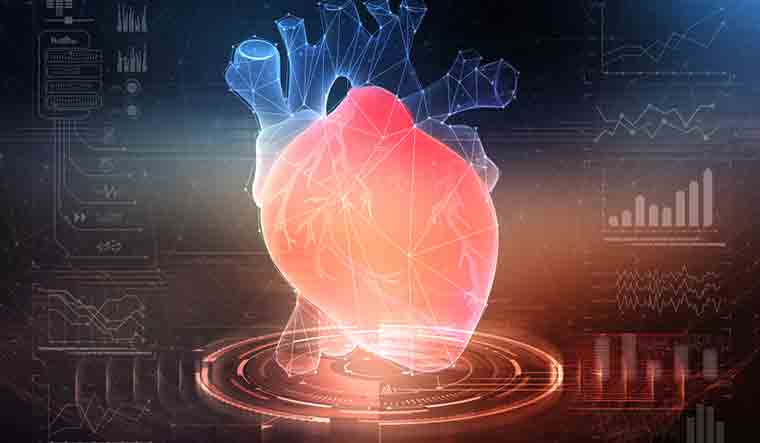The image depicts a computer-generated, medical-style illustration of a human heart, prominently displayed at the center. The heart is detailed in varying shades of pink and coral red, with its arteries, aorta, and other ventricles rendered in a light blue, all presenting geometric patterns and a semi-transparent quality. The background is primarily black, adorned with an array of dimly-lit circuitry and graphs, including pie charts, line graphs resembling heartbeat traces, and other chart types in white or light gray. The human heart is perched atop a glowing, digitized, bright orange disc, adding to the futuristic and holographic aesthetic of the image. The overall composition suggests it could serve as a sophisticated backdrop on electronic devices, blending medical visualization with high-tech design elements.